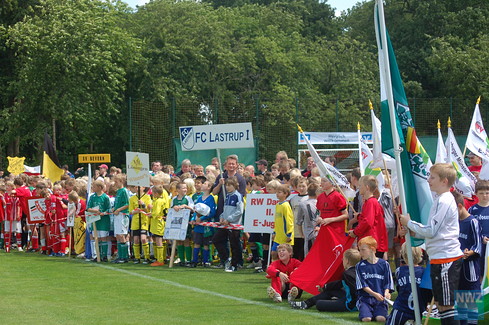This image captures a lively children's soccer event held on a green, grassy field marked with white painted lines. The participants, likely aged 9 to 12, are from various teams, each distinctively clothed in red, green, yellow, blue, and combinations thereof, with some donning black shorts. The scene is vibrant with children holding up large flags and signs, suggesting a celebratory or competitive gathering. A notable sign reads "FC Last Rupp One," indicating a possible team name or event title. The backdrop includes a tall green fence and a picturesque array of green trees, all under a bright daytime sky. Numerous adults are present, possibly coaches or supporters, adding to the festive atmosphere of the event.